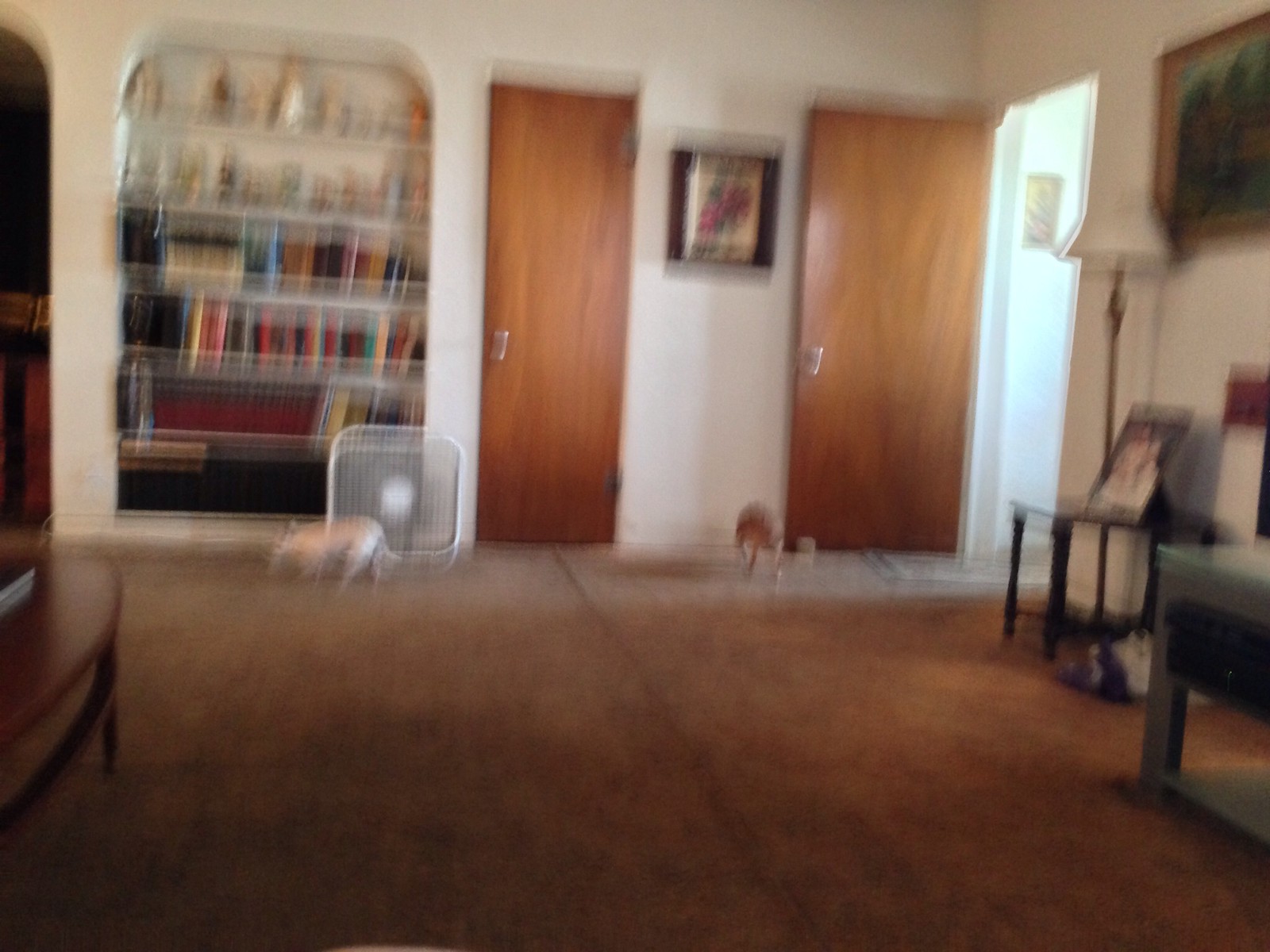In this grainy and highly blurred indoor photograph, taken from a low angle as if the viewer is seated on the floor, the scene appears to be within a cozy home or apartment. The floor is covered with brown linoleum, adding a warm, retro touch to the setting. Dominating the upper right corner, an open door reveals a white wall outside, signifying a connecting room. The doors to the right and left are of a stained brown wood, each adorned with a silver hardware handle, contributing to the room's modest, lived-in charm.

Positioned in the upper left corner of the image, a built-in shelf area is visible on a white wall. The central shelves are filled with books, suggesting a love for reading or a home library. The top two shelves hold various objects, which appear to be small statues, though their details are lost to the blur. Adjacent to this shelf, a dark, indistinct shape is seen pressed against the wall.

On the lower right side of the photograph, there are two tables. One table has an object leaning against it, possibly a framed photograph. The other table is mostly out of the frame, with only its legs and a corner visible, hinting at a gray color. The overall atmosphere of the image, despite its blurriness, evokes a sense of everyday comfort and personal space.